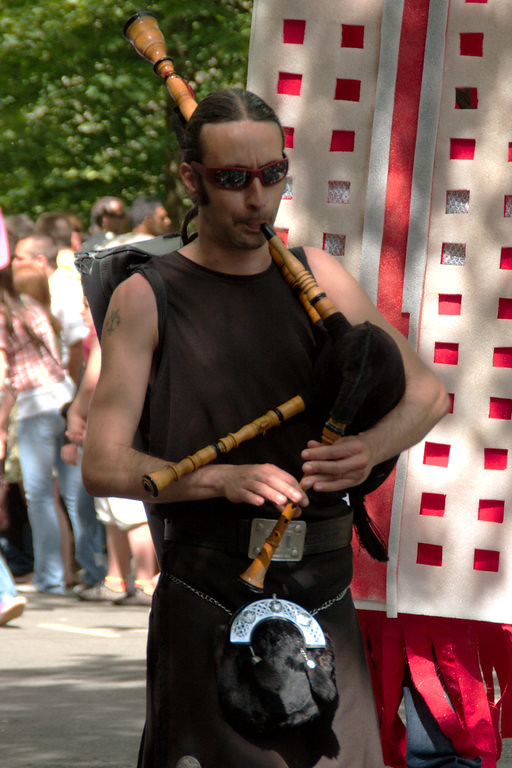In this vibrant outdoor scene, a man is the centerpiece as he passionately plays the bagpipes. He is dressed in a striking black tank top coupled with a matching black kilt, complete with a silver belt adorned with the traditional furry sporran. His long dark brown hair is secured in a ponytail, and he sports dark sunglasses with bright frames that add a touch of flair. The bagpipes he plays are distinctive with their brown wooden pipes and a black bag. The scene is festive, with a possible indication of a renaissance fair or parade, further suggested by the red and white decorative awning and the red ribbons beneath it. Behind him stands a cream-colored structure with a grid-like design and red paper accents. Crowds of people are milling about in the background, hinting at a well-attended event. The sunlight filters through green trees on the left, enhancing the joyful and lively atmosphere of the gathering.